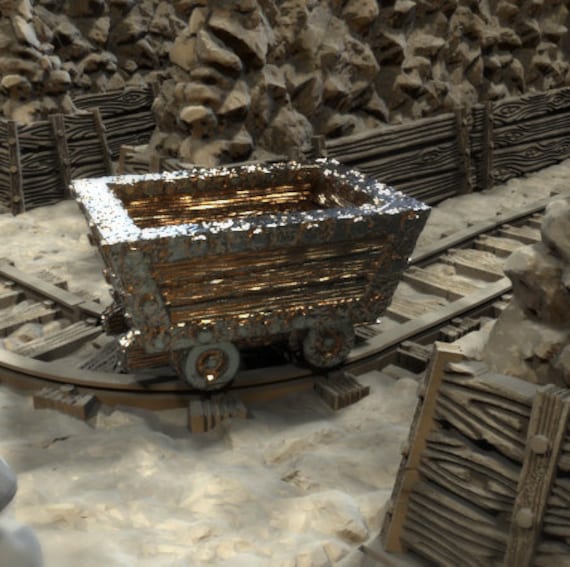This close-up photograph, taken indoors in a museum-like setting, captures a meticulously crafted 1/16th scale model of a historic mining cart. Set against a square, four-inch by four-inch backdrop, the image reveals intricate details of the cart and its surroundings. The mining cart, positioned in the center, features gleaming gold and silver accents; the side panels are adorned with shiny gold plating, while the metal frame combines both gold and silver elements, diverging from the dull wood and metal typical of authentic mining equipment.

The cart, reminiscent of those used to transport minerals like coal, iron ore, gold, and silver, rests on a curved section of railroad track. The track winds through a simulated mine environment, with light brown and gray dirt scattered around. Four silver wheels support the cart, which resembles a bucket designed to be loaded and pushed along the tracks.

Surrounding the track, the scene includes realistic details such as wooden retainer walls buttressing the overhead rocks to prevent them from sliding. A small rock formation with a board atop it is visible in the lower right corner, emphasizing the rugged terrain. Although stylized with decorative gold and silver, the scene captures the essence of a historical mining operation, making it an intriguing exhibit piece within a museum display.